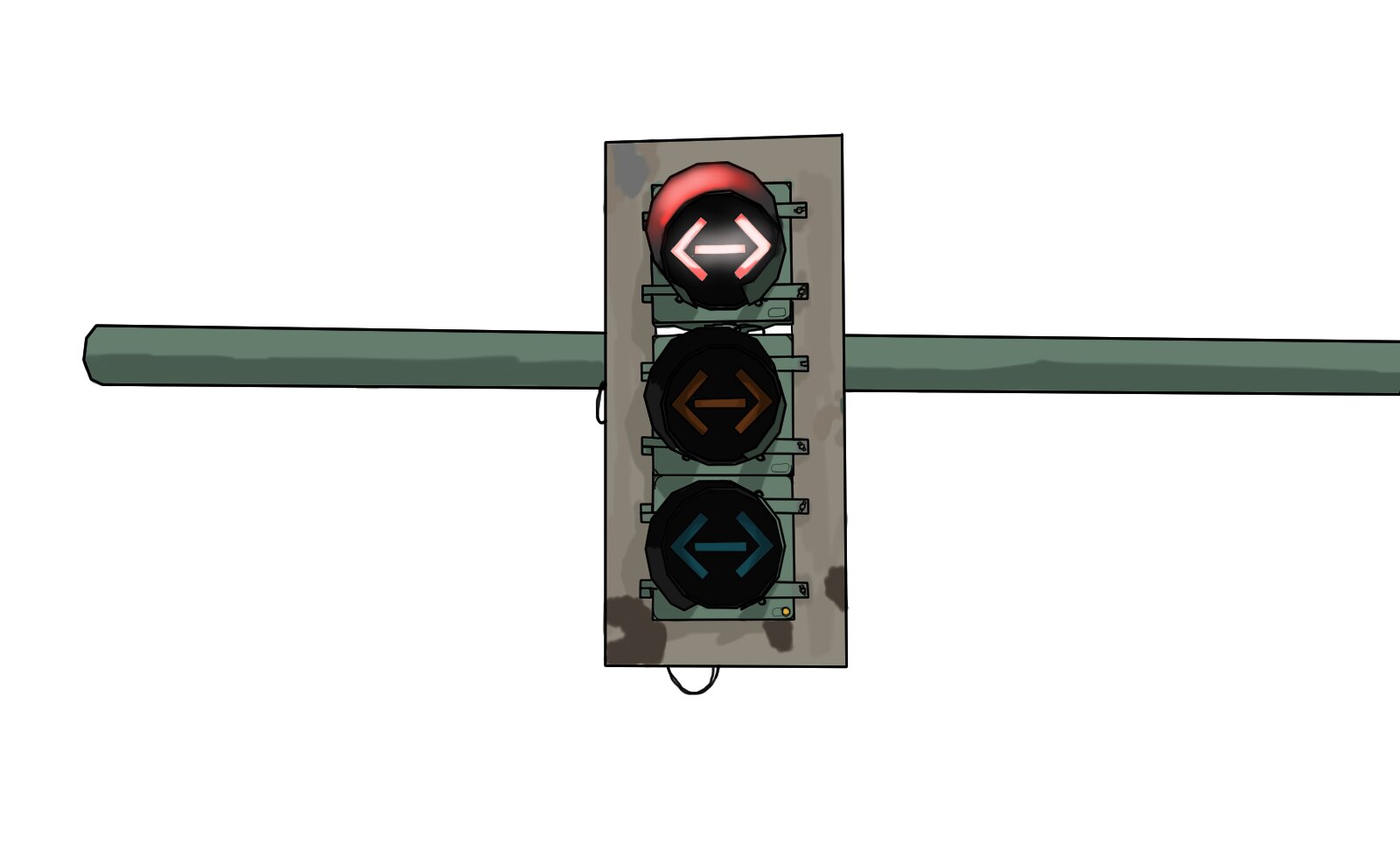This is a computer-generated illustration of a modern traffic light system with an artful twist, akin to an anime style or comic book drawing. The image features a horizontal bar, blending silver and green hues, extending across the entire width of the picture. At the center of this bar is a vertical, rectangular traffic light housing that is an intriguing mix of silver, grayish-green, and slightly splotchy brown textures.

The traffic light itself features three circular lights mounted vertically: red at the top, yellow in the middle, and green at the bottom. Unusually, each light displays a symbol rather than a solid color. The symbol consists of a horizontal dash flanked by double-ended arrows pointing left and right, resembling a less-than, dash, greater-than sequence (<- ->). In the illustration, the red light is currently lit, illuminating the symbol in red, while the yellow and green lights, though not lit, share the same symbolic design.

Additional details include a U-shaped black wire hanging from the bottom of the traffic light, complemented by a smaller wire protruding from the left side of the vertical housing. The background is a stark white, which accentuates the colors and details of the traffic light system.